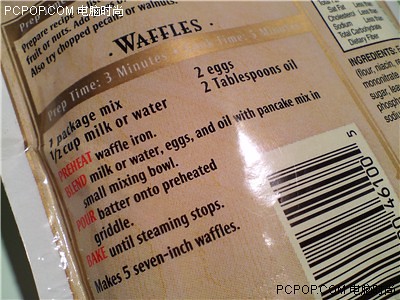This image showcases the back of a light brown food package for a waffle mix, captured at a slight angle tilting towards the bottom left. The package is bordered in white and features detailed cooking instructions and ingredient lists. In a gold rectangle, it indicates "Prep time, three minutes." Below this in black text, the ingredients needed are: one package mix, 1 1⁄2 cup milk or water, two eggs, and two tablespoons of oil. The instructions are clearly outlined; "Preheat" (in red text) a waffle iron, "Blend" (in red text) milk or water, eggs, and oil with the pancake mix in a small mixing bowl, pour batter onto the preheated griddle, and bake until steaming stops. The recipe yields five seven-inch waffles. A barcode is present to the right of the text, placed sideways, and a black and white design with various numbers at the bottom. Additionally, in the upper left corner of the image, there's a text overlay that reads PCPOP.com and some Chinese characters, suggesting a possible origin or branding detail.